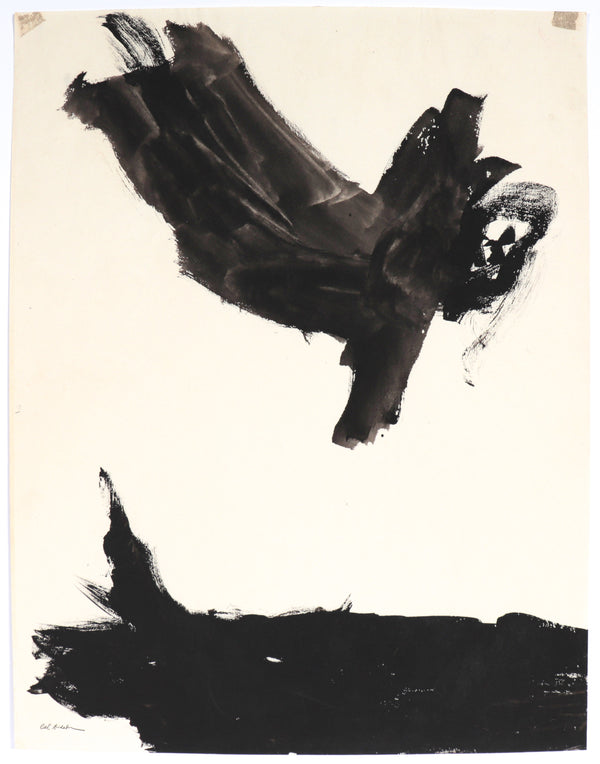This painting features an abstract composition rendered in black paint on a light background that appears predominantly grayish white with hints of pink. The background is textured, suggesting some depth, with lighter hues at the bottom transitioning to a slightly deeper tone towards the top. The artwork primarily consists of bold black brushstrokes that form intriguing patterns and shapes across the canvas.

At the bottom of the piece, a significant horizontal black brushstroke extends nearly the entire width of the canvas, with a notable upward curl on the left side, resembling a wave or splash of water. This bottom stroke leaves intermittent gaps where the background color peeks through, adding texture and dimension.

Towards the middle to upper portion of the canvas, a striking black smear descends diagonally from the upper left corner toward the right, broadening into a vertical slash that appears almost like a crude depiction of an object or figure. This area also features additional black squiggles and smudges to its right, creating a complex interplay of forms.

Moreover, at the top corners of the painting, there are small square-like areas that appear slightly different, possibly indicating remnants of tape or some other material that was once adhered there but has since been removed.

The artwork, reminiscent of a child’s playful creation or a spontaneous abstract experiment, is signed in an illegible scrawl at the bottom left corner, adding a personal touch to this evocative and interpretive piece.